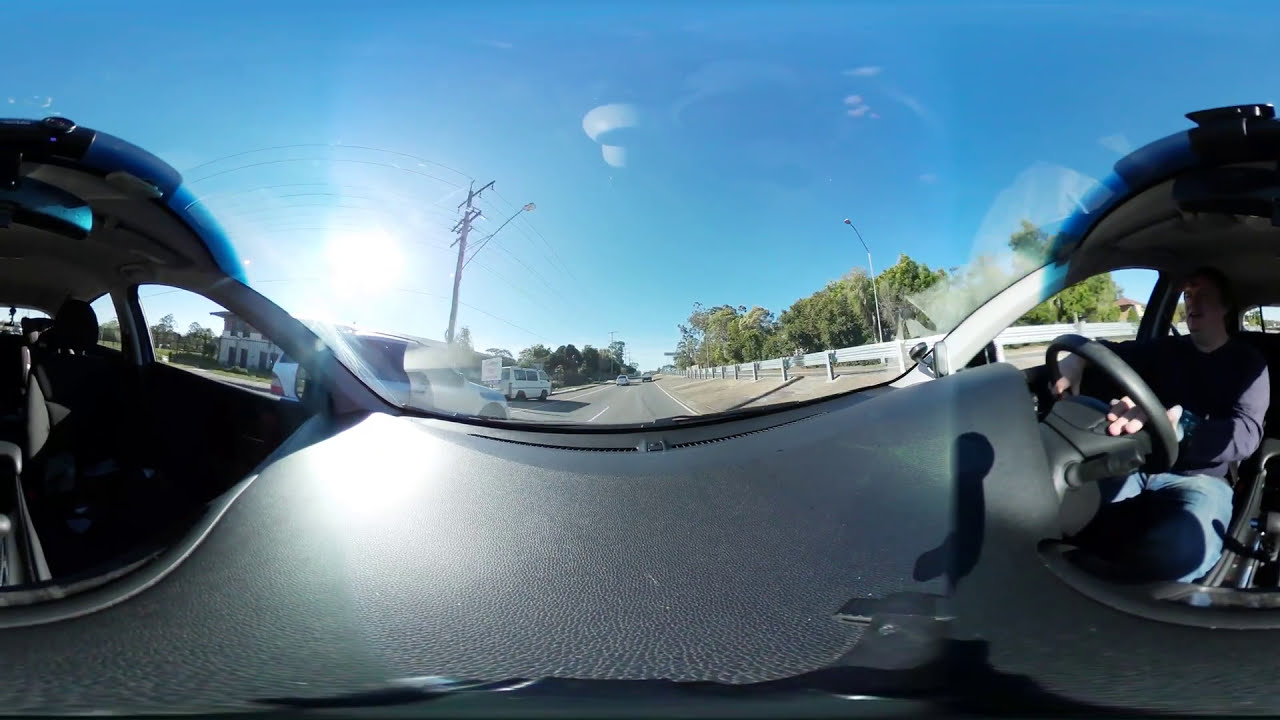This is a 360-degree panoramic image taken from a dash-mounted camera inside a car, showing a distorted view that includes both the driver and the passenger sides. The driver, a white man wearing a dark long-sleeve shirt and jeans, is on the right side of the image, gripping the steering wheel with both hands. His darkish hair is clearly visible. The dashboard is situated in the center of the image, featuring the windshield and wipers, with a view of a three-lane road ahead. The road has light traffic, including some cars and a van. On the left side of the image, you can see the empty black passenger seat and through its window, a two-story building and electrical posts with wires. The blue sky, with a few scattered white clouds, forms the picturesque backdrop, and the sun is glaring brightly on the left side of the image, near the electric lines. The right side of the road is lined with trees, street lamps, and a metal guardrail that runs alongside a fence and another building visible through the driver’s window.